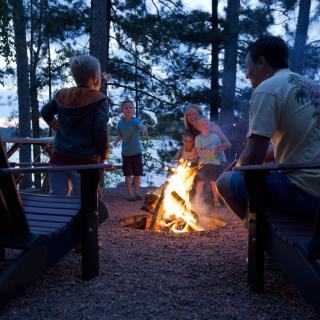In this detailed family photo, a mom, dad, and their four children, aged between roughly four to ten, are gathered around a large campfire. They are surrounded by a picturesque forest setting, with mature pine trees and a serene lake in the background. The scene unfolds on a dirt ground, indicating a natural camping experience. 

The family is comfortably seated on Adirondack chairs, perfect for their outdoor gathering. The dad, wearing a white shirt with a graphic on the back, is seen on the right-hand side, intently staring at the fire. Standing next to his chair, his son shares the same fascination with the flames. The mom, smiling warmly, is crouched over holding two of the younger children on her lap, while a fourth child in a blue shirt points excitedly at the fire. 

The overall mood is joyous and relaxed, captured around sunset, transitioning into night, as the image is relatively dark. The warmth of the fire illuminates their happy faces while they roast marshmallows, dressed in short sleeves and shorts, suggesting a warm and pleasant evening. This scene beautifully encapsulates the essence of a lovely family vacation in the great outdoors.